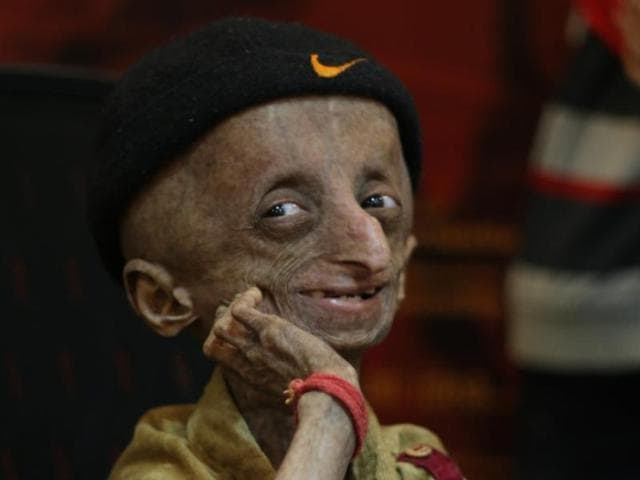The photograph is a color image in landscape orientation, capturing a young man known as Nihal Bitla, who has a genetic disorder causing him to appear much older than he actually is. Positioned slightly to the left but centrally framed, Nihal's face shows a big smile as he gazes up to the left, his chin propped on his right hand. His skin is dark and splotched with wrinkles, and he has a curved nose and sparse eyebrows. He wears a black Nike cap featuring a yellow logo on the front, a beige shirt with a maroon patch on the left shoulder, and a red cloth bracelet on his right wrist. The background is blurred, displaying indistinct black, white, reddish, and bluish shapes, adding to the focus on Nihal's expressive face. The overall image is bright, clear, and detailed, capturing the complex and unique appearance of the young man against an abstract backdrop.